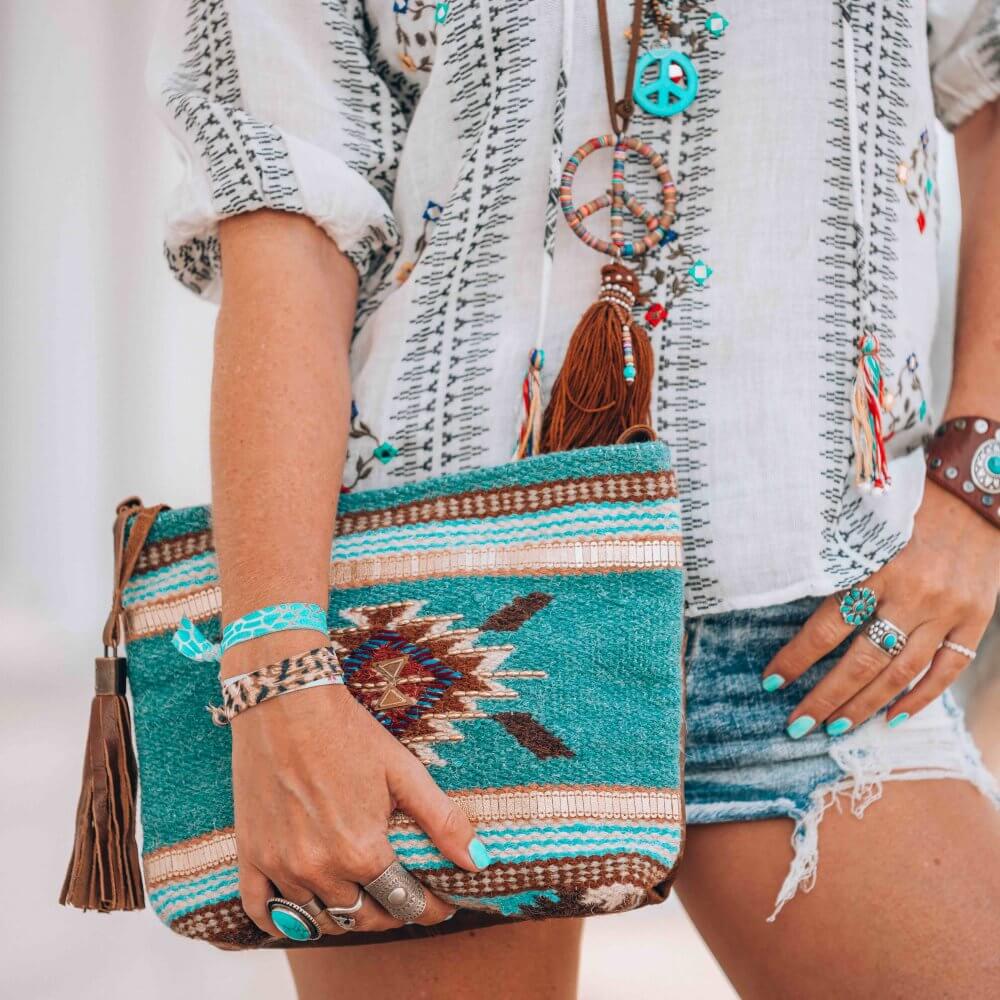The image depicts a bohemian-styled woman from her chest to her thighs. She is carrying a small, multi-colored bag that features black, blue, white, brown, and light brown hues and is positioned on her right hip. The bag has a retro vibe, reminiscent of the 60s and 70s, and appears to be made from cloth, though one description mentions it being made of wood. She is dressed in a white T-shirt decorated with vertical black designs and wears jean miniskirt. Her ensemble includes multiple necklaces with peace symbols and other bohemian designs, turquoise being a prominent color throughout her accessories. She sports several wristbands on both hands; the ones on her right hand are green and white, brown and black, and an additional white band, while her left wrist has a larger, brown wristband. She also wears various rings—one with a blue stone, another gray—and her fingernails are painted turquoise. The scene is brightly lit, suggesting it is photographed outside against a white background.